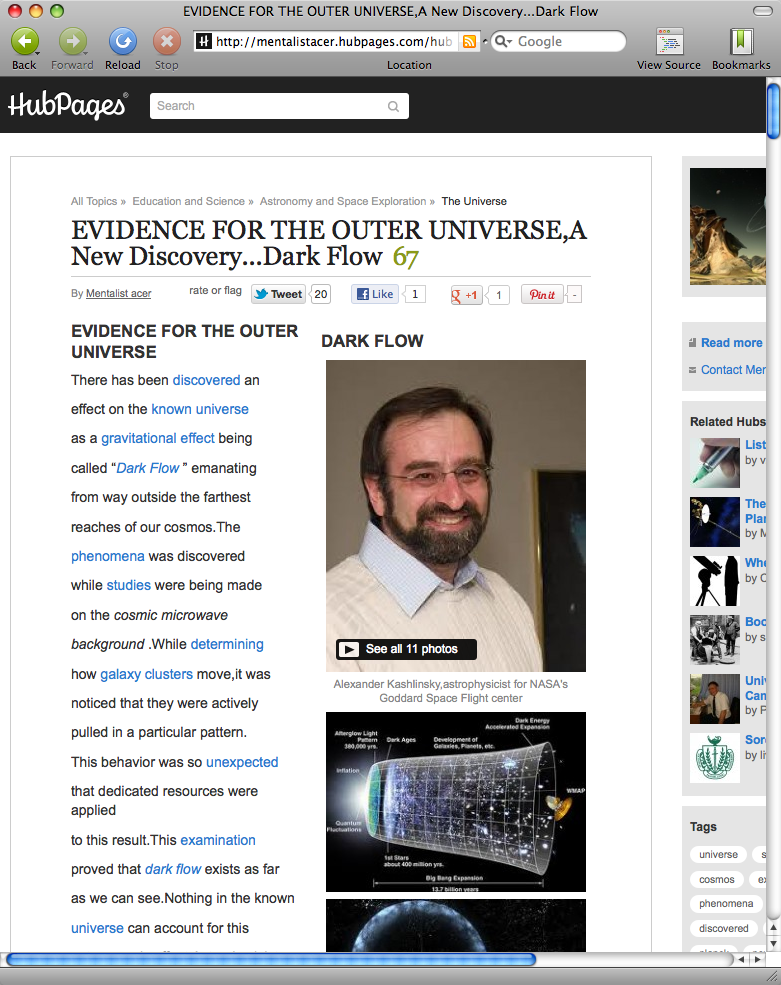Screenshot displaying a webpage from a mobile browser

At the top of the screenshot, there's a gray navigation bar. In the upper left corner, there are three small circles in red, yellow, and green. The navigation bar also includes a series of buttons: back, forward, reload, and stop. Following these buttons is a search bar containing a website URL, and a Google search bar is visible to its right.

Below this navigation bar, there is a black header area labeled "HubPages" in white text, which includes an additional search bar. The primary content area of the screenshot features what appears to be an article titled "Evidence for the Outer Universe: A New Discovery.... Dark Flow" with a green number "67" next to the title.

Within the body of the article, rows of black and blue text are visible. To the right of the textual content, there is an image of a man. He has black hair, a black mustache, and a black beard. He is wearing glasses, a blue button-up shirt, and what appears to be a white sweater. Beneath this image, text identifies the man as Alexander Kovarsky and states that he works for NASA's Space Flight Center.